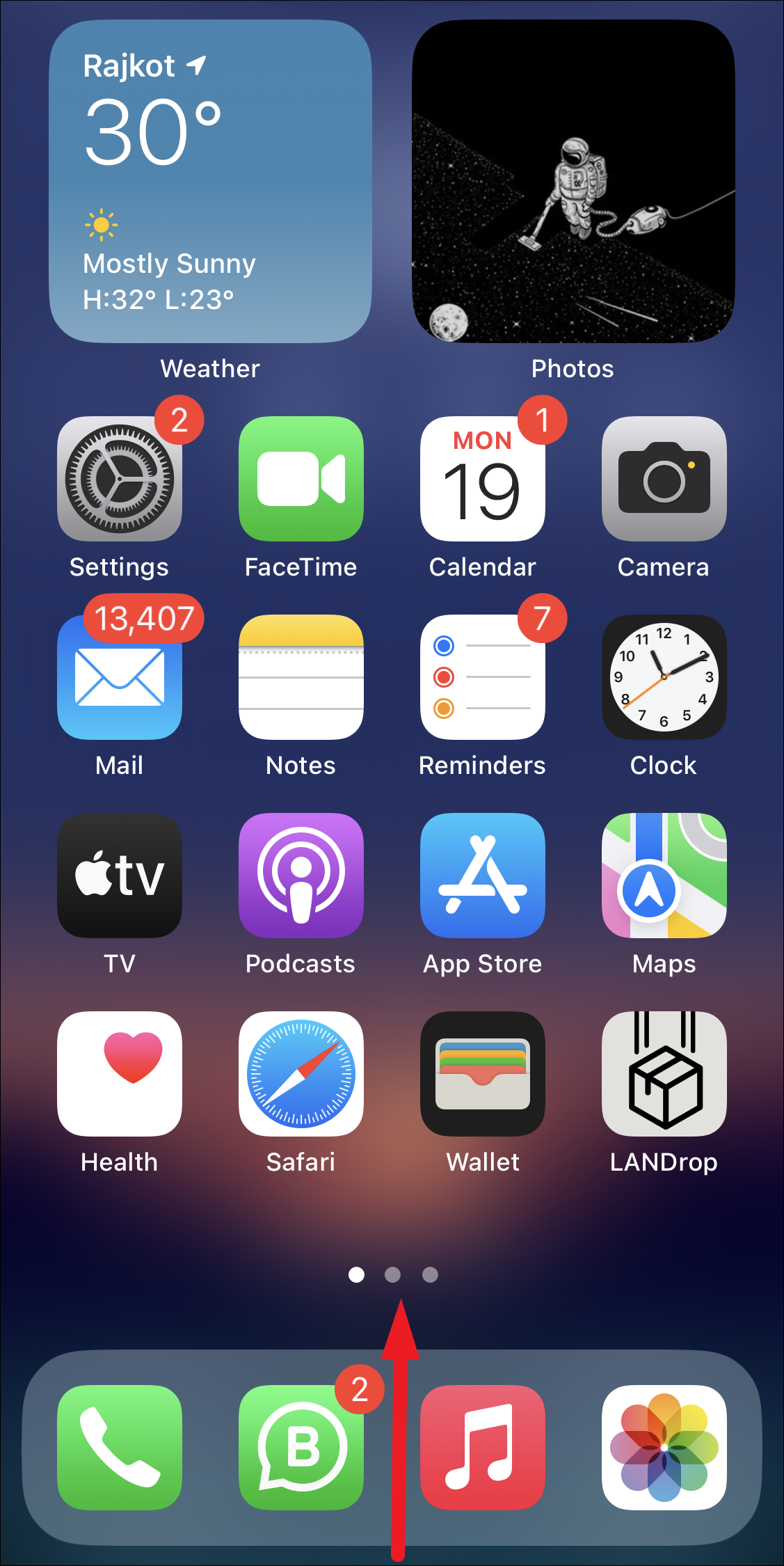This image is a detailed screenshot of the home screen of an Apple device, likely an iPhone or iPad, as suggested by the presence of Apple symbols and icons. At the top of the screen, there is a weather widget displaying the current conditions in Rajkot, showing a temperature of 30 degrees Celsius, described as mostly sunny, with a high of 32 degrees and a low of 23 degrees.

To the right of the weather widget is a photo widget featuring an amusing image of an astronaut sweeping up dirt with a vacuum in space. Below these widgets, familiar app icons are arranged in a grid layout. The icons include: Settings, FaceTime, Calendar, Camera, and Mail, the latter showing a staggering 13,407 unread emails, highlighting the owner's busy schedule. Other apps displayed are Notes, Reminders, Clock, TV, Podcasts, App Store, Maps, Health, Safari, Wallet, and AirDrop.

At the bottom of the home screen, the dock contains four frequently used app icons: the Phone app, an icon labeled with the letter 'B' and a number 2, the Music app symbol for Apple Music, and the Photos app for accessing the device's gallery. This comprehensive layout provides a snapshot of the user's digital life, organized yet bustling with activity.